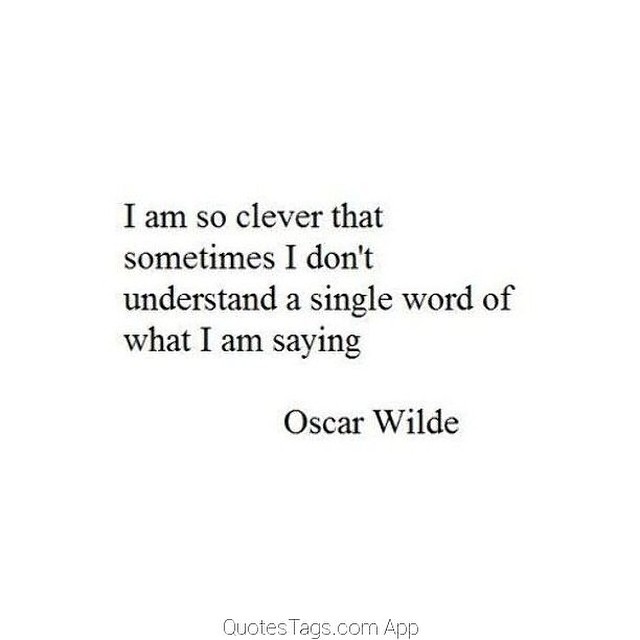The image features black text on a white background, originating from the Quotetags.com app, as indicated by a logo at the bottom. The quote prominently displayed in a font resembling Times New Roman reads: "I am so clever that sometimes I don't understand a single word of what I am saying." This quote is arranged in four distinct lines to evoke the appearance of a poem. Below the quote, the name of the author, Oscar Wilde, is also written in black text without any punctuation.